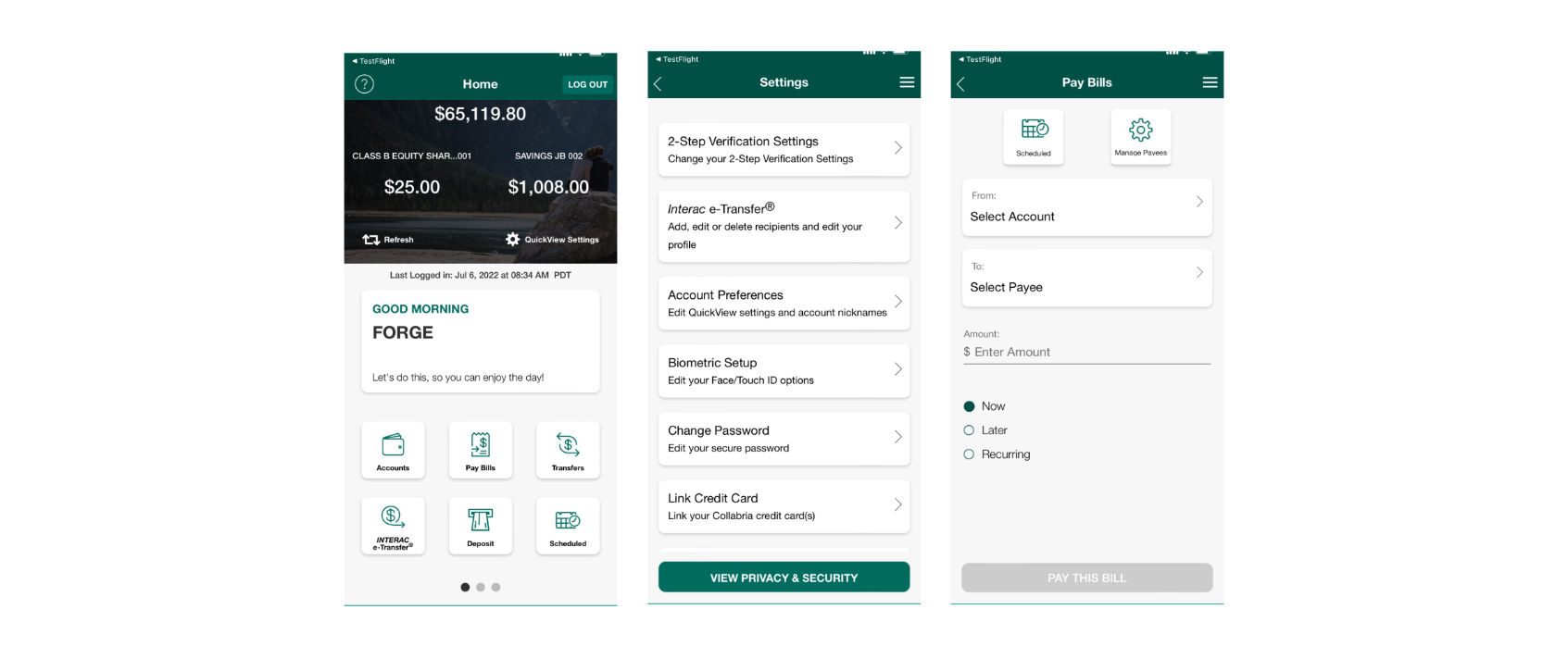Here is the revised and detailed caption:

---

The image showcases three screenshots from a comprehensive mobile banking app, each highlighting different key functionalities.

1. **Home Screen**: The first screenshot presents the home screen where the user has a balance of $65,000, along with a welcoming message, "Good morning Forge, let's do this. Enjoy your day." The navigation bar at the bottom features six quick access icons: Accounts, Pay Bills, Transfers, Interac e-Transfer, Deposit, and Schedule, facilitating easy navigation through the app.

2. **Settings Screen**: The second screenshot delves into the settings menu, detailing various options for enhancing account security and customization. It includes enabling two-step verification, managing Interac e-Transfer preferences, configuring account settings, setting up biometric authentication (such as Face ID or Touch ID), changing passwords, linking credit cards, and accessing privacy and security options.

3. **Bill Payment Screen**: The third screenshot depicts the bill payment interface, offering users the flexibility to navigate and pay bills immediately, schedule them for later, or set up recurring payments. This functionality streamlines the process of managing finances directly within the app.

Together, these screenshots provide a detailed overview of the app's primary functions, which include account management, enhancing security settings, and facilitating bill payments. This mobile banking app aims to simplify financial management and ensure users can efficiently handle their banking needs all in one place.